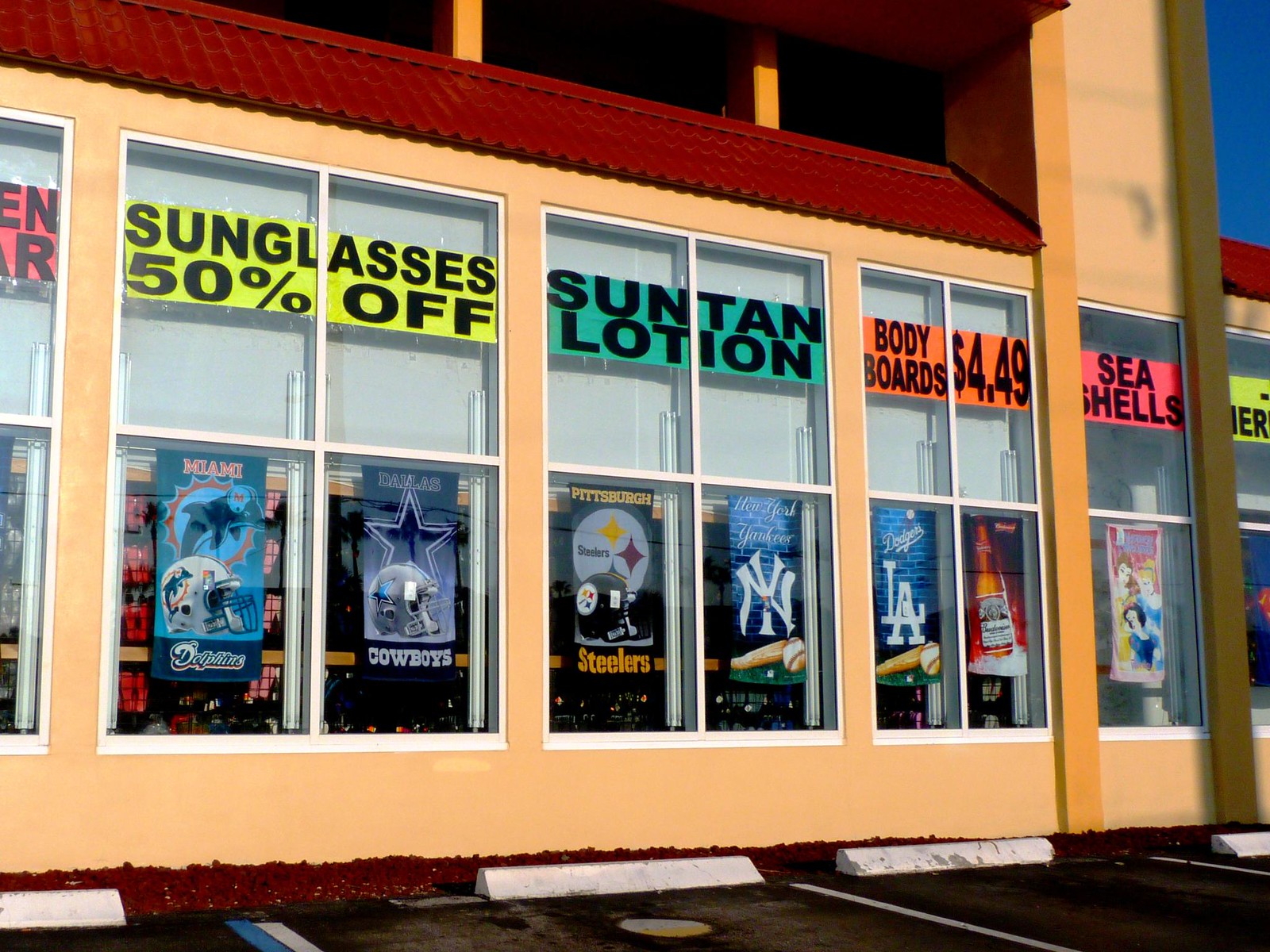This color photo captures the exterior of a beachside souvenir shop, likely a Super Wings or similar store. The building features a slanted, clay tile-like roof in a reddish-brown shade, supported by tan pillars. The primary facade is tan with large windows framed in white. These windows display colorful banners advertising sales: a bright yellow banner with "Sunglasses 50% off" in black font, a turquoise blue banner promoting suntan lotion, an orange banner offering body boards for $4.99, and a hot pink banner for seashells.

Below these banners, the windows showcase an array of NFL and MLB-themed beach towels, including teams such as the Miami Dolphins, Dallas Cowboys, Pittsburgh Steelers, New York Yankees, and LA Dodgers. There's also a Disney princess towel, though no Cincinnati Bengals representation is visible. Additional advertisements include a bottle of Budweiser and various sports teams’ paraphernalia.

The surroundings feature a newly paved black asphalt parking lot with gray bumpers to prevent vehicles from hitting the building, clearly marked parking spaces, and a designated handicap space. The scene is set against a backdrop of a clear blue sky, enhancing the attractive and inviting atmosphere typical of a beach souvenir shop.